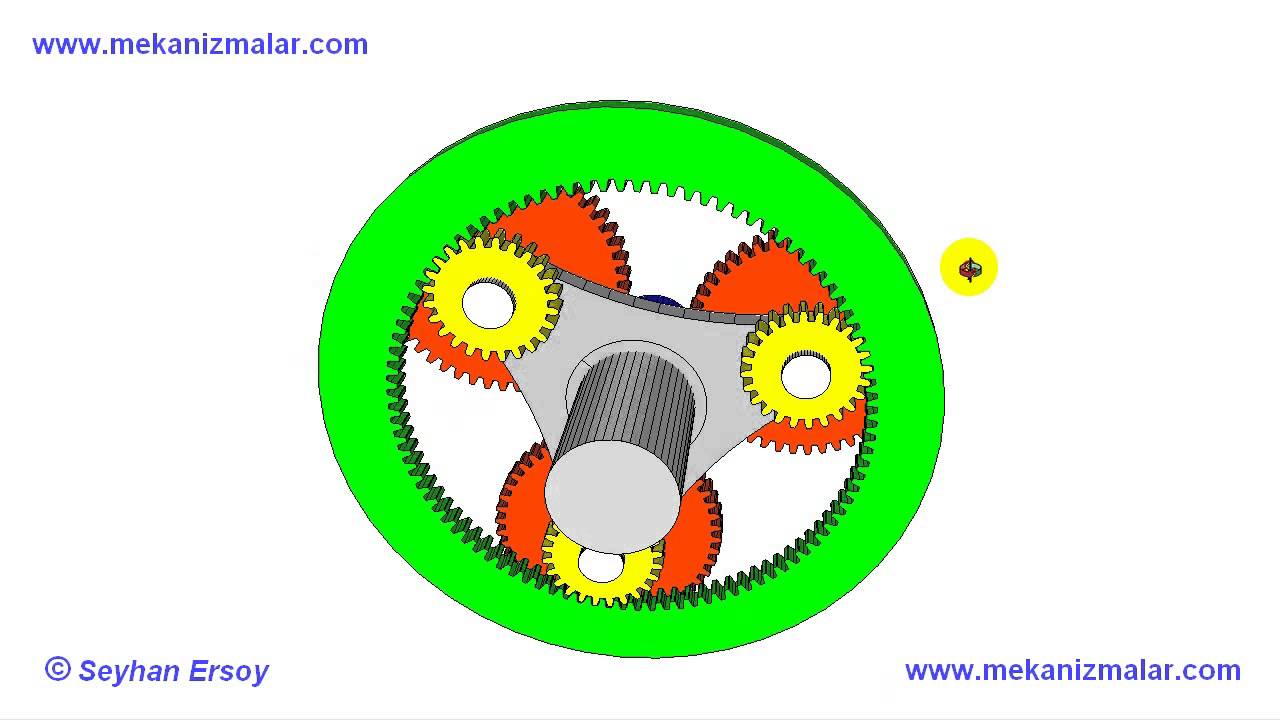This image features a detailed, computer-generated diagram of interconnected gears on a white background. At the core of the diagram is a prominent bright green gear, characterized by teeth along its inner edge. This large gear is linked to three medium-sized red gears, which are positioned at the corners of a metallic, triangular piece. This triangular component has a handle or knob at its center, displaying intricate striations. Each red gear is further connected to an outer smaller yellow gear, placed at the corners of the triangle, ensuring a synchronized motion when the knob is turned. The primary colors in the diagram include electric green, taxicab yellow, and red, with additional metallic silver and white elements.

Text details in blue font include the website "www.mechanizimir.com" located twice, once in the top left corner and once in the bottom right corner. Additionally, the bottom left corner bears the name "Sehan Ersoy."